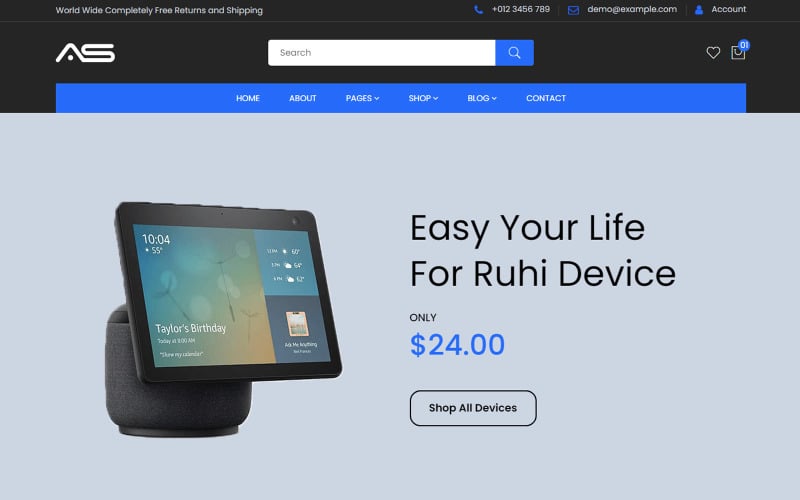This image is a detailed screenshot of a website, showcasing various interactive elements and a product advertisement prominently. At the top of the page, a black banner spans the width of the screen, containing blue and white text. The black banner features essential navigational and contact information: a telephone icon followed by a phone number, and an envelope icon with an email address, both presented in white font. A white search box labeled "search" in gray letters, accompanied by a small magnifying glass icon within a blue rectangle, is situated to the right.

Directly beneath the search functionality, a horizontal blue navigation bar displays key website sections in white text: "Home," "About," "Pages," "Shop," "Blog," and "Contact." 

The focal point of the image is an advertisement for a device—a tablet speaker. The ad showcases the product with the text: "Easy your life for Ruhi device, only $24" written adjacent to the image of the device. The price "$24" is highlighted in blue. Below the advertisement, a black-outlined oval contains the black text "Shop All Devices," inviting users to explore more products. A small outlined heart, rendered in a thin white line, is also visible, potentially serving as a wishlist or favorites indicator.